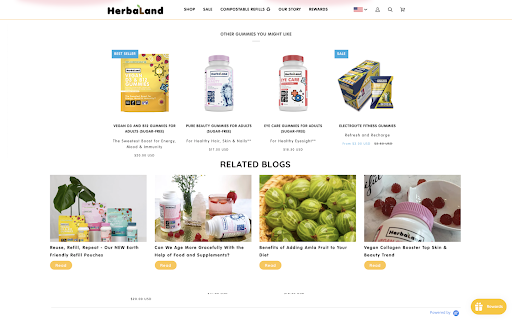This image is a screenshot of a store website named "Herbatland" (H-E-R-B-A-L-A-N-D), showcasing their homepage. At the top of the page, there's a bold banner menu displaying navigational links including "Shop," what appears to be "Sale," and "Our Story," followed by "Rewards." Additionally, there's an American flag as a dropdown option, presumably for selecting different languages. The top-right section of the banner features icons for user account access (represented by a head and shoulder icon), a search function, and a shopping cart.

Below the banner, there's a partially visible message that starts with "Check," though the complete text is unclear. The main content area displays a grid of four product images. The first image on the left shows a yellow box; the next two images in the middle appear to be pillboxes, and the fourth image on the right depicts another box, which seemingly contains a smaller container within it. Due to the small size of the screenshots, specific text and details on the product images are difficult to discern.